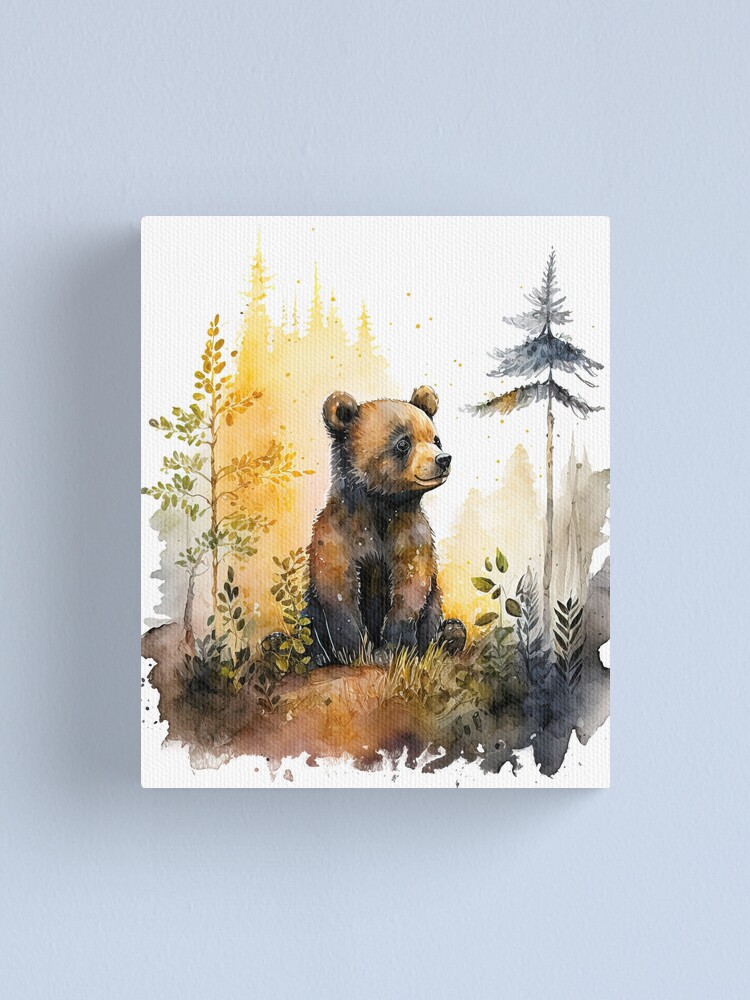This image features a detailed watercolor painting of a baby bear positioned at the center of a square white canvas, which is mounted on a light blue wall. The baby bear, depicted with rich textures, has a dark brown torso and lighter brown face where the sunlight touches, accentuating its youthful innocence. With expressive dark eyes, a black nose, and a lighter tan muzzle, the bear looks slightly to the right. Seated on sandy-brown, grassy ground, its front paws rest vertically on the ground while one hind leg is visible.

Flanking the bear are variations of trees and vegetation. To the right, an evergreen with a tall, slender trunk and sparse branches towers over the scene. To the left, there is a lighter green tree with more foliage, and there are additional dried grasses and small bushes scattered around. The background of the canvas is primarily white with subtle, softly painted areas of orange and gray, suggesting sunlight and depth. Surrounding the painting is a faint, blue-hued backdrop, and scattered paint splatters add an abstract element to the scene. The overall color palette consists of earthy browns, light greens, and hints of yellow and orange, giving the painting a warm and serene atmosphere.